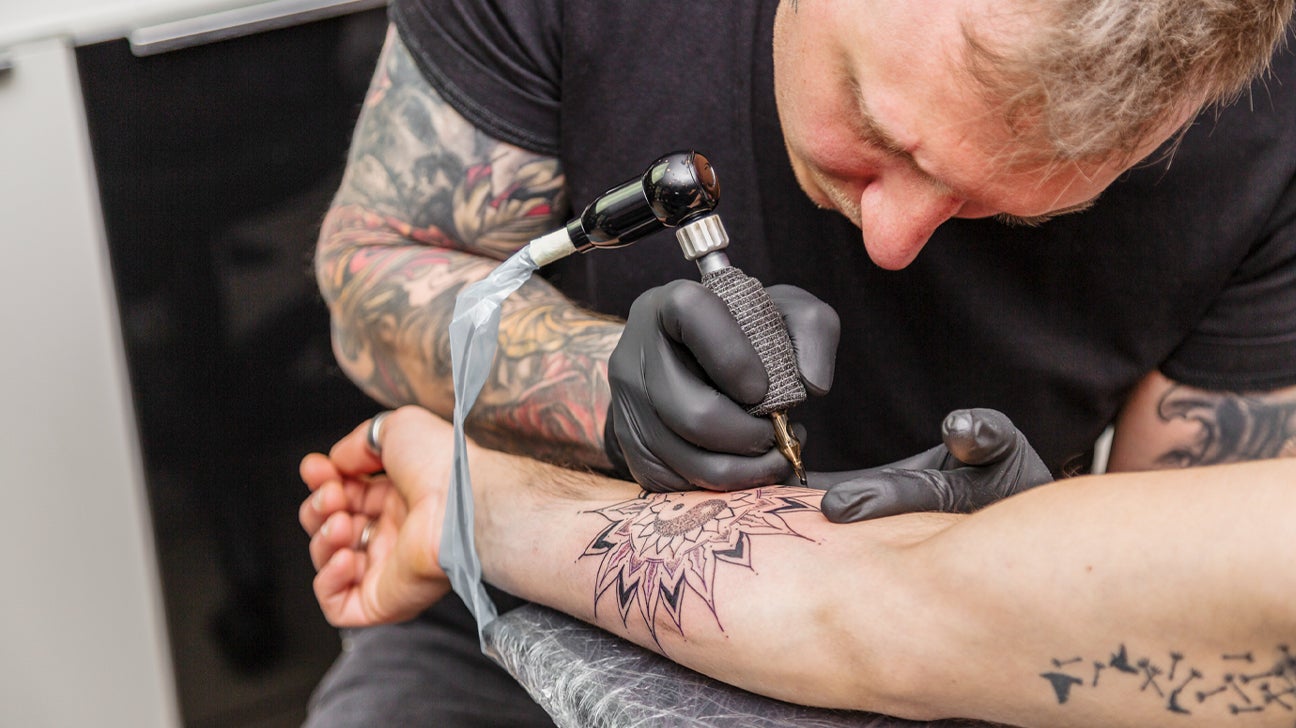In this detailed photograph, a tattoo artist with thinning blonde hair and a mustache intently focuses on his work, tattooing a large, intricate flower design with a yin-yang symbol in the center on a client's forearm. The scene is set in a tattoo parlor, with the artist, dressed in a black t-shirt and dark grey gloves, wielding a tattoo gun. Both the tattoo artist and the client, who extends his arm from the bottom right to the left of the image, have numerous existing tattoos. The client's arm, adorned with artwork including what appears to be a nail-like design on the inner bicep, also features noticeable dark arm hair near the wrist. Additionally, the client sports a thumb ring and a simple silver band on their middle finger. The grey and white table supports the client's arm, which extends off the edge, creating a clear stage for the detailed tattooing process.